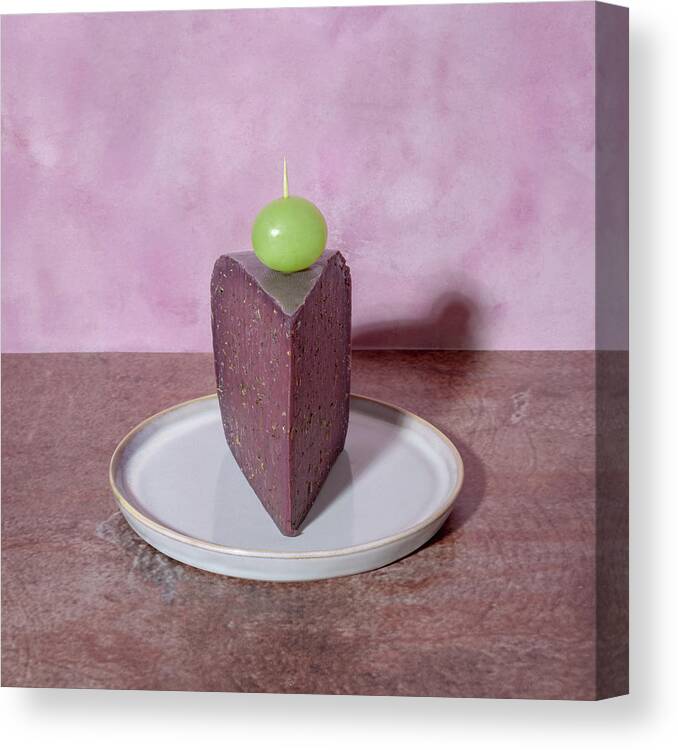A detailed canvas portrait features a slender triangular slice of purple-colored cake, possibly cheesecake, or cheese with various colored flecks and hints of brown. This intriguing piece of food is topped with a perfect round green grape, secured in place with a toothpick. The cake sits on a small, flat white dish with subtle yellow detailing around the edges. The dish rests atop a wooden table with a purplish hue. The background of the image is a light pink to purple tone, adding a soft contrast to the overall composition. The detailed texture and color variations in the food make this an appetizing and visually engaging image.